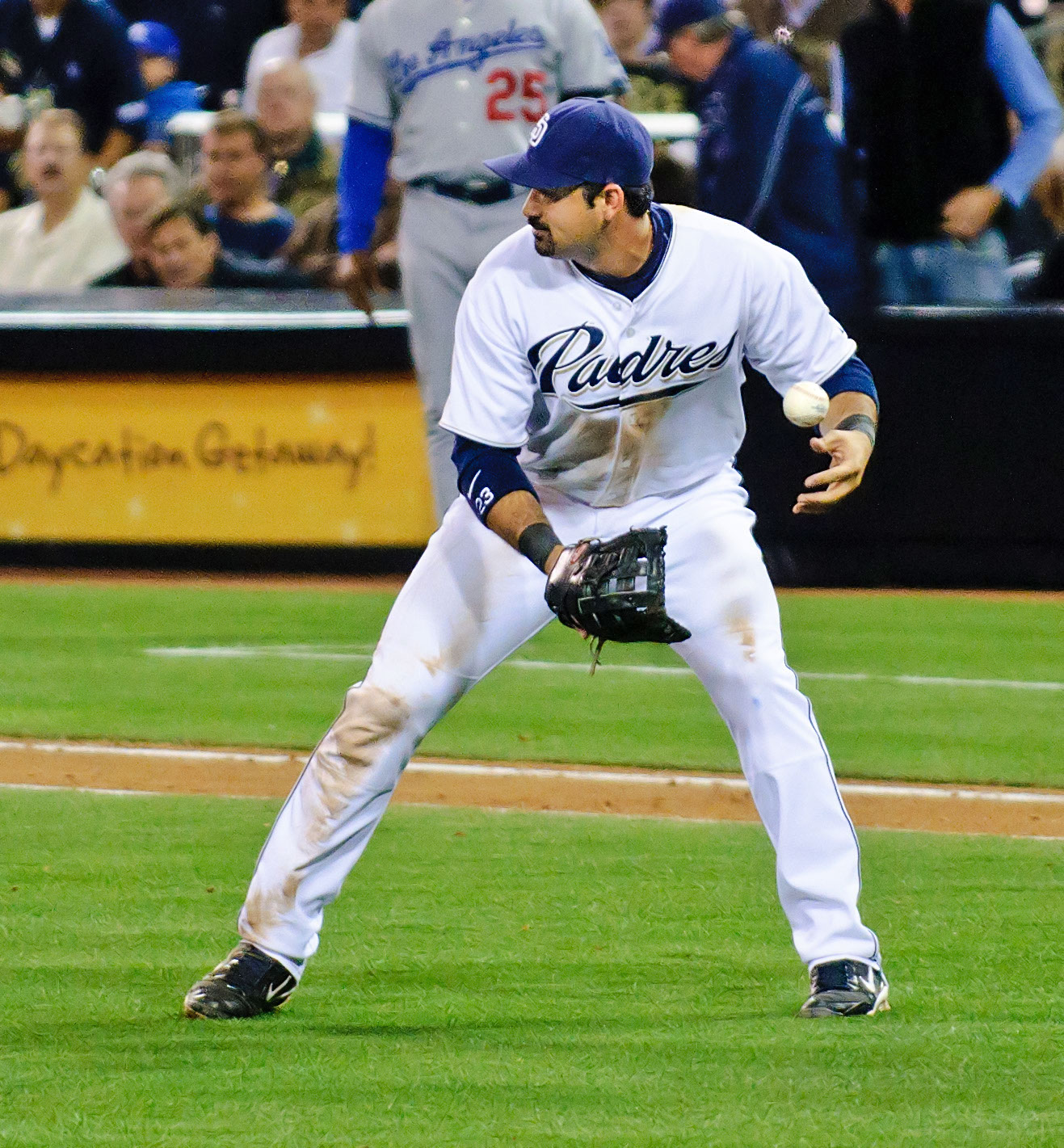This image captures a professional baseball player from the San Diego Padres in a dynamic moment on the field. The player, presumably Adrian Gonzalez, is in full Padres uniform, consisting of a white short-sleeve jersey with "Padres" written in dark blue cursive across the chest and white pants—all streaked with dirt, suggesting recent action. He wears a long-sleeve blue undershirt, a black wristband marked with the number 23, black cleats featuring a white Nike swoosh, and a dark blue cap with a white "SD" logo. The player is standing in profile, with his black glove ready and a baseball inexplicably suspended midair just above his left hand, indicating a possible error or a trick play moment. His stance and attention are directed toward home plate. The background reveals blurry spectators in the stands, a yellow advertisement on the wall, and details of the infield, including the first baseline with white chalk. Notably, a Dodgers coach, distinguishable in a gray uniform with "Los Angeles" and the number 25 in red, is visible behind him, hinting at a game against the Los Angeles Dodgers.